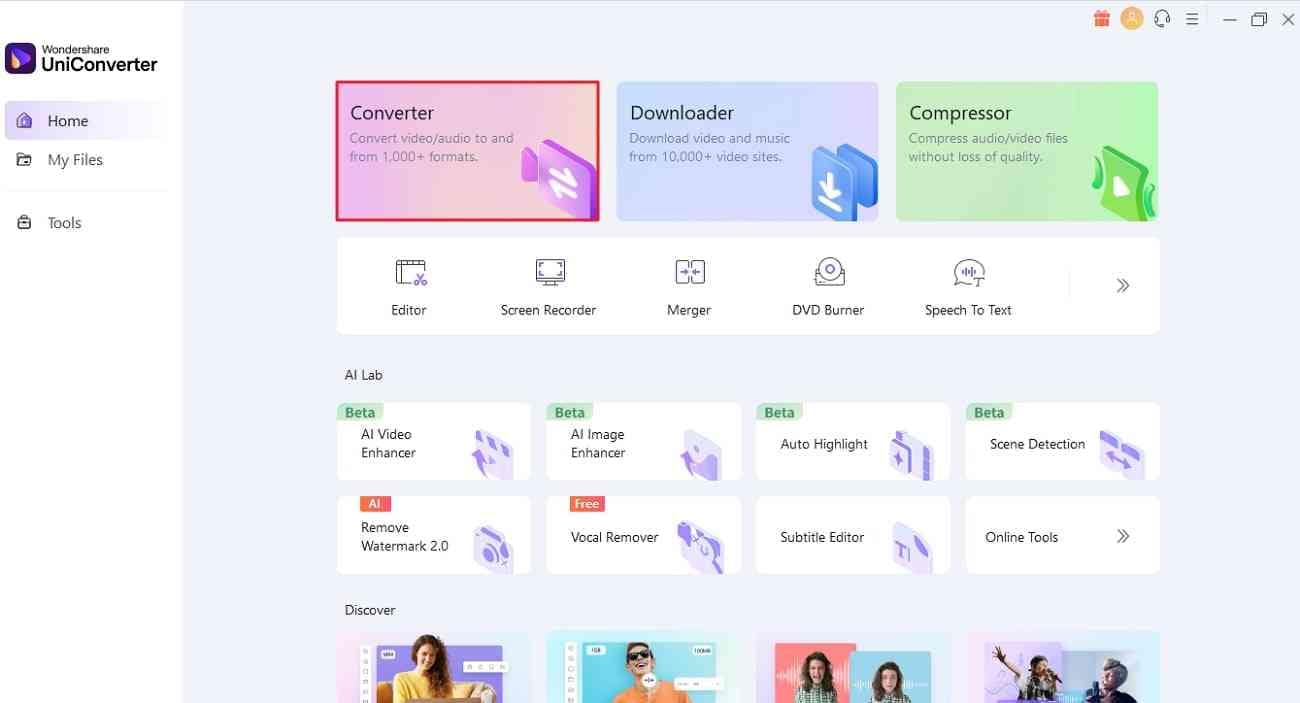Screenshot of Wondershare UniConverter Homepage

The image showcases a screenshot of the Wondershare UniConverter application homepage. Dominating the top section, "Wondershare UniConverter" is prominently displayed beside a unique 3D curved logo with contrasting yellow and purple hues housed within a purple square.

On the left sidebar, there are navigation options labeled "Home," "My Files," and "Tools," each accompanied by respective icons: a home icon, a folder, and a toolbox.

In the main content area, three colored panels provide an overview of the core functionalities:

1. **Converter** - Displayed in a pink box, this section highlights the ability to convert video and audio files to and from over 1,000 formats. It is symbolized by a pink icon featuring arrows pointing in both directions.

2. **Downloader** - Set in a blue box, this area emphasizes the feature of downloading video and music from over 10,000 video sites. It is represented by a blue icon with a download arrow.

3. **Compressor** - Shown in a green box, this part focuses on compressing audio and video files without a loss of quality. The green icon depicts a play button being warped from both sides.

Below these core features, there is an array of five icons related to various utilities: 
- Editor
- Screen Recorder
- Merger
- DVD Burner
- Speech to Text

An arrow indicates additional features can be accessed.

Further down, an "AI Lab" encompasses four sections, each marked as beta and offering advanced capabilities: 
- AI Video Enhancer
- AI Image Enhancer
- Auto Highlight
- Scene Detection

Underneath, there are more AI-driven features like:
- AI Remove Watermark 2.0
- Vocal Remover
- Subtitle Editor

Additionally, a segment for "Online Tools" is present.

At the very bottom, a "Discovery" section includes four photographic examples showcasing before-and-after enhancements performed within the application, demonstrating various editing and enhancing techniques.

This detailed interface overview illustrates the extensive functionalities offered by Wondershare UniConverter, designed to cater to various multimedia processing needs.